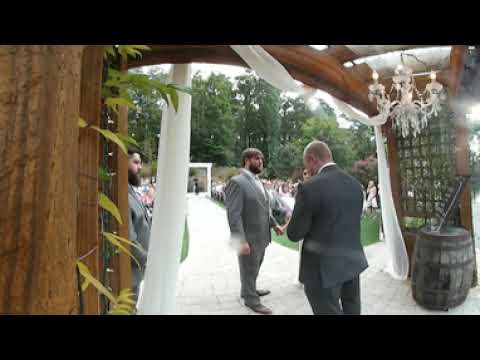The image captures a serene outdoor wedding ceremony, framed by a charming brown wooden gazebo decorated with veils, vines, and a chandelier hanging from the roof on the right side. Central to the image is the minister, seen from behind wearing a grey suit and white shirt, with light hair cropped close to his head, looking downwards. The groom, also in a grey suit but in a lighter shade, sporting a full beard and brown hair, is standing opposite the minister, tenderly holding the hand of his bride. Partially obscured by the minister, the bride's face and white dress peek into view. Next to the groom, likely the best man, another gentleman in a grey suit with a long beard stands. At the minister's feet stretches a white walkway, possibly ceramic tiles, lined with guests seated on both sides. To the right, a brown whiskey barrel adds rustic charm, and the background reveals a lush line of dark green trees visible past a white arch. The scene is set in a grassy area, captured in a low-resolution but rich in intimate details, beautifully preserving the moment of union amidst nature.